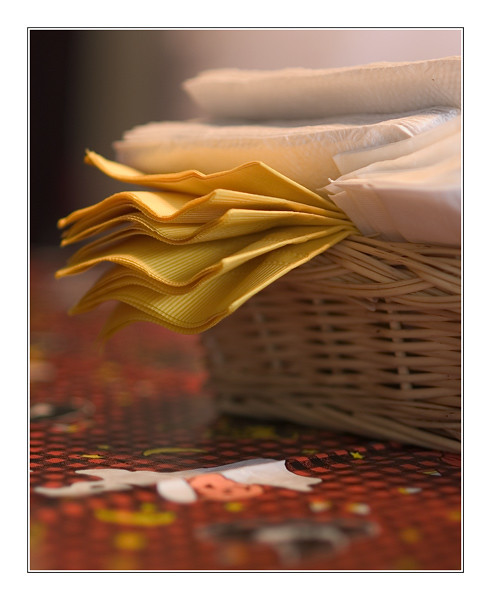The image showcases a close-up photograph centered around a light tan wicker basket holding a mix of napkins. The basket sits prominently towards the center and slightly to the right of the frame, with its right edge partially cropped out of the image. Inside the basket is a stack of white textured napkins, visible mainly toward the top and rightmost part of the basket. Draped over the edges of the basket are five silky, fine dining-style yellow napkins, cascading down the center and center-left side. The basket rests on a decorative tablecloth featuring a striking pattern of red and black crisscrosses. The background of the image is out of focus, creating a bokeh effect that blends black, white, and gray hues, with black dominating the top left, white on the right, and gray around the center left. The overall aesthetic hints at an autumn or Halloween theme, with subtle, undiscernible shapes and faces possibly suggesting festive motifs.